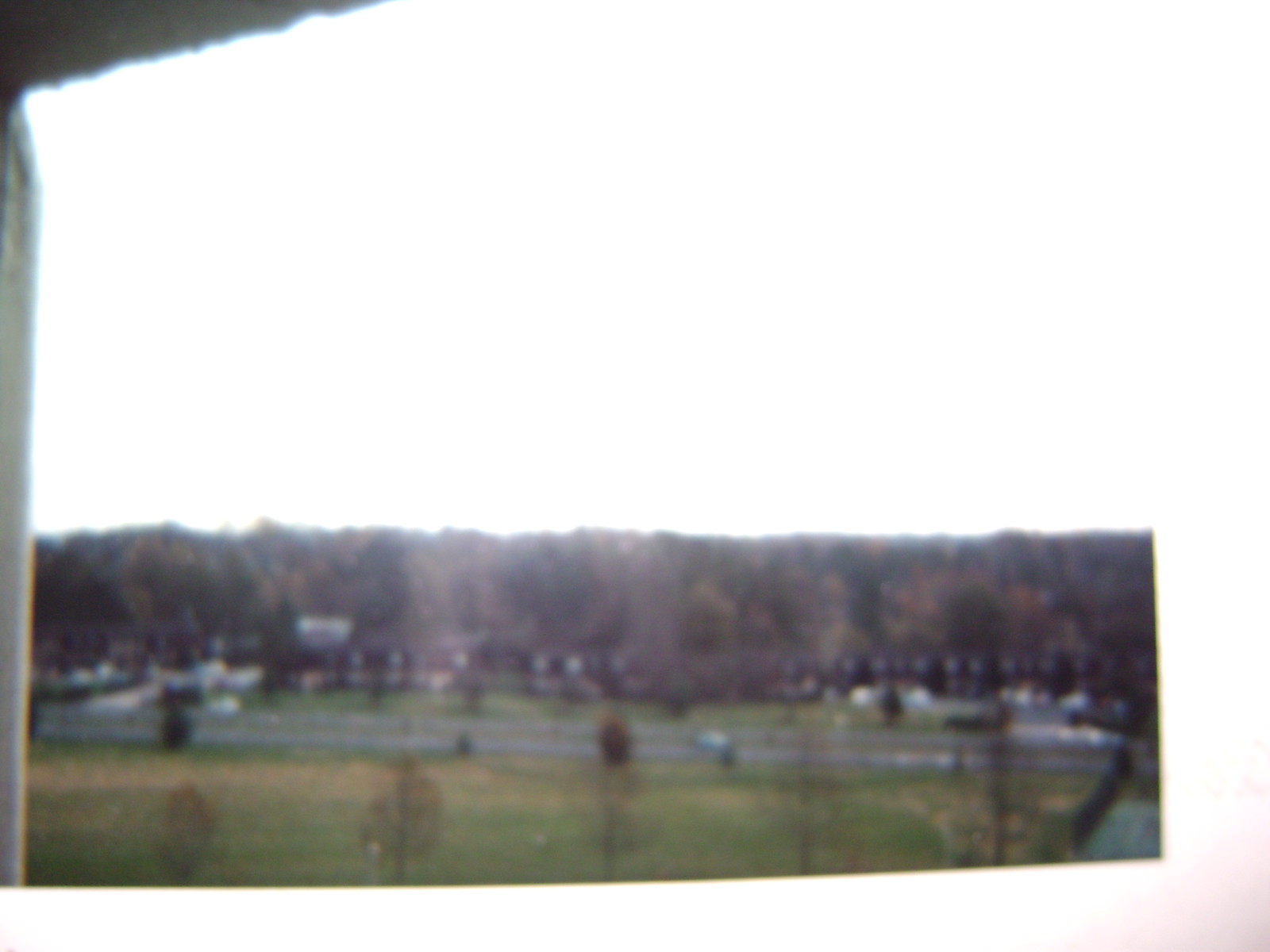The image shows a grainy, blurry photo taken from inside, looking out of a large window partially framed by a curtain on the left side. The scene outside features a large grassy area in the foreground, tinged slightly brown on the left. A row of mostly leafless trees stretches across the image, with at least one visible red tree towards the center bottom, indicating a touch of fall. Behind these trees, there is a suggestion of a long row of townhomes or similar houses, identified by their brown rooftops and lighter lower sections. Two windows are visible in the roof area of these buildings. A road runs in front of these buildings, where a small blue vehicle is faintly discernible on the right. The background showcases a densely wooded area filled with tall, bare trees, giving way to a bright white sky occupying the top part of the image. The picture itself appears discolored, possibly pinkish at the edges, and shows signs of being an old, poorly focused photograph with some light glare.